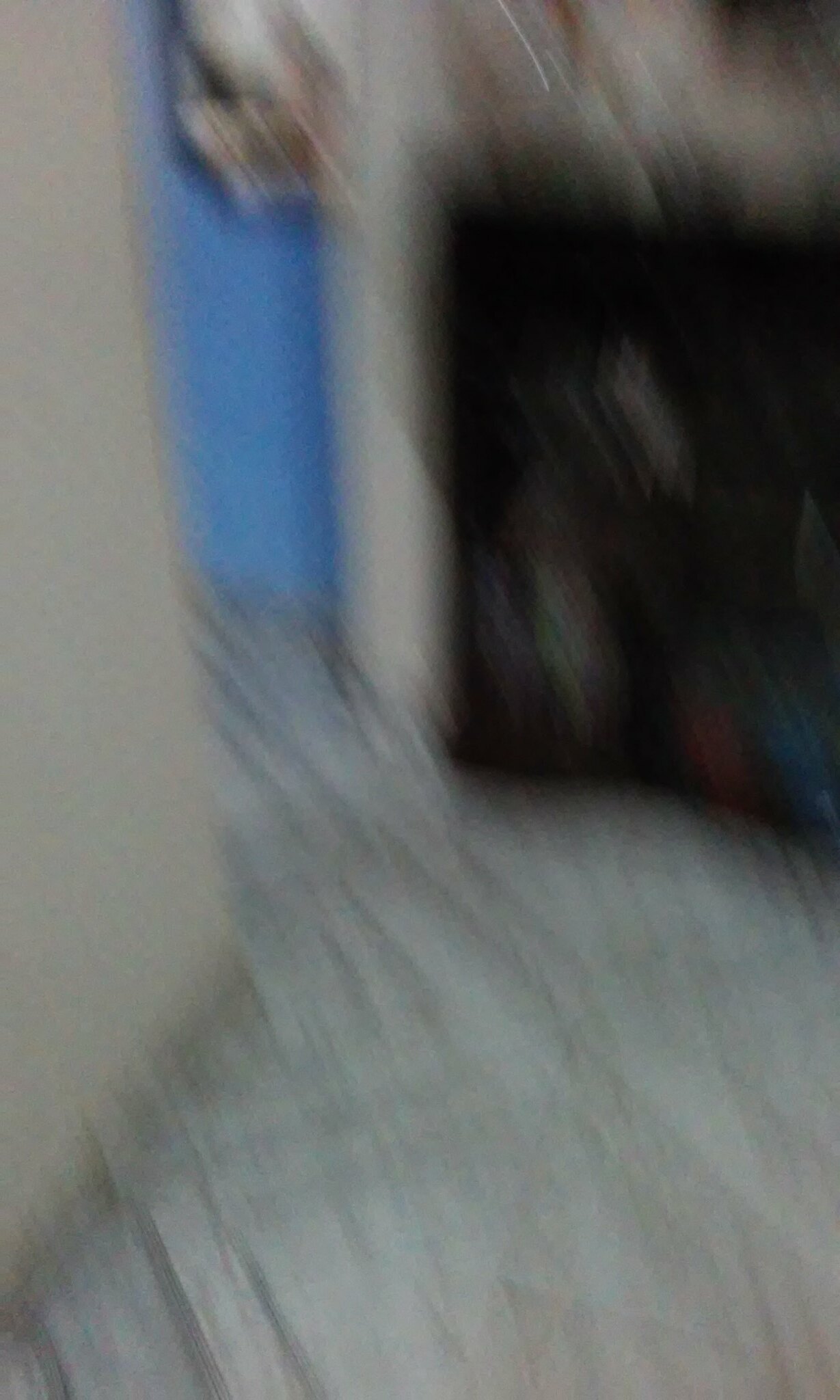The image is quite blurry, making it difficult to discern specific details. However, it appears to depict a room with a visible floor and a wall with a doorway on the left side. Just in front of the doorway stands what seems to be a wooden cabinet. Through the doorway, a blue wall is visible with a white object hanging on it. The floor appears to be covered with a white tapestry.